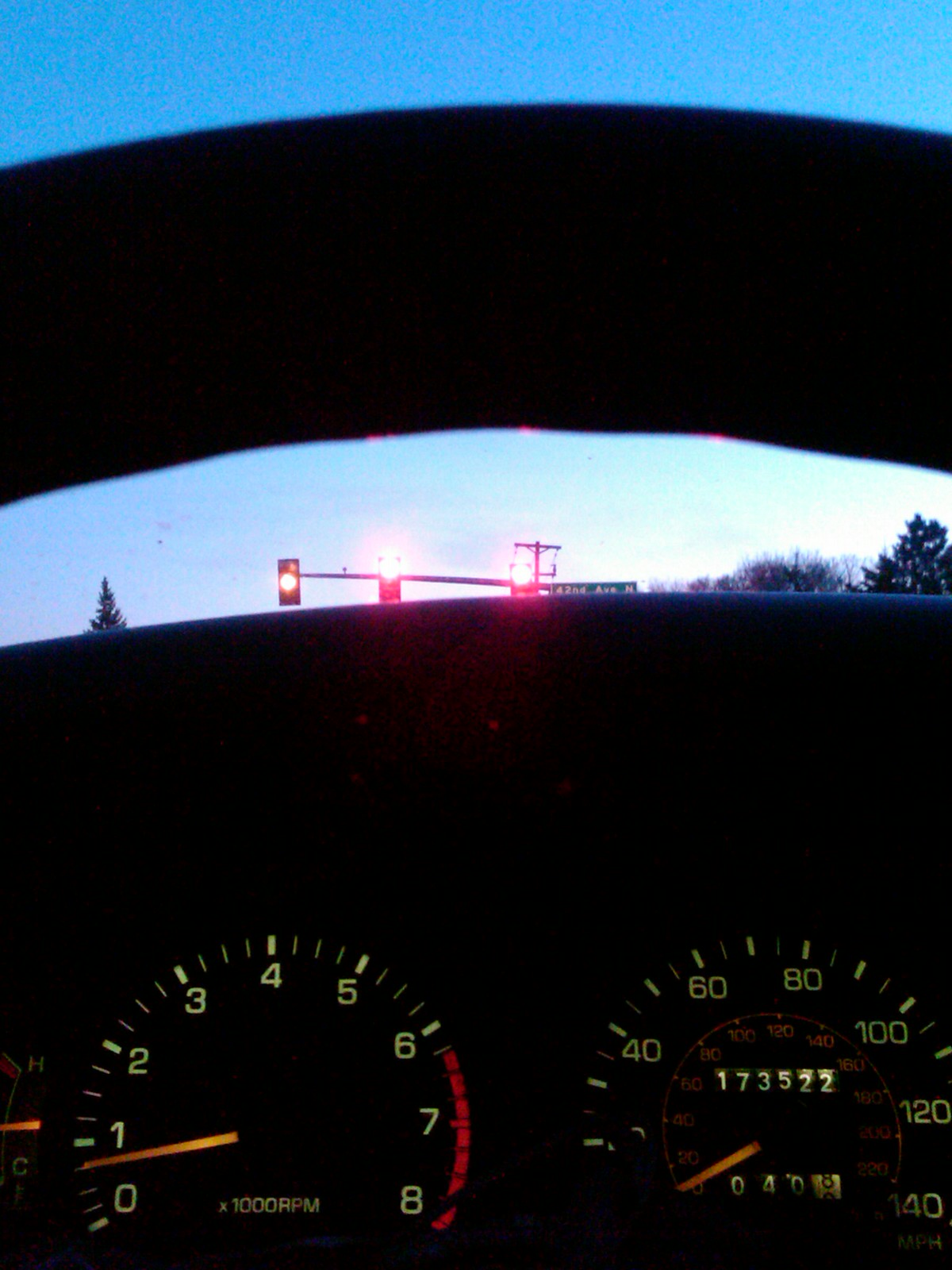The image features a detailed close-up of a car dashboard with various instruments prominently displayed. On the far left is a round heat dial. Next to it is a tachometer, with the needle resting below 1,000 RPM, indicating an idle engine. To the right of the tachometer, the speedometer reads zero, showing the car is stationary. The speedometer also contains an inner ring displaying the car's mileage, which is 173,522 miles, and the trip odometer, which reads over 400 miles. Visible at the top of the image is the steering wheel's upper arc. Beyond the dashboard, outside the car, a traffic light is visible. The traffic light has two red signals for the straight and right-turn lanes and a yellow signal for the left-turn lane. The scene outside the car includes a blue sky with scattered white clouds and the tops of a few trees. This clear daylight scene, captured in the background, hints at an early time of day with light just above the horizon.